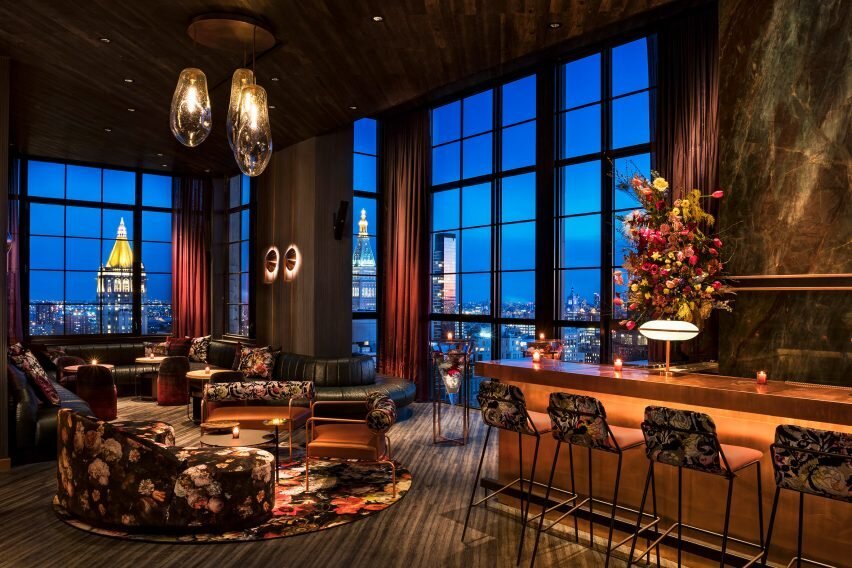This image showcases a sophisticated lounge area, potentially in a high-rise restaurant or hotel lobby, offering a stunning view of a city's skyline through floor-to-ceiling windows adorned with long, flowing drapes. On the right side, there's an elegant bar with four brown floral print chairs, illuminated by three votive candles and a beautiful light centerpiece surrounded by a grand floral arrangement. Adjacent to the bar is a luxurious seating area featuring a wraparound dark gray leather sofa, paired with a mix of matching floral print and round low-to-the-floor chairs set around small round tables with candles. The room is dressed in stylish design elements, including striped rugs, teardrop pendant lights hanging from the ceiling, and two large, quirky "googly eye" motifs on the wall. The deep blue evening sky and city lights, including a distinctive lit-up building with a pointy top, add to the ambiance of this high-altitude, elegant setting. The intricate details and coordinated patterns create a refined atmosphere perfect for social gatherings and relaxation.